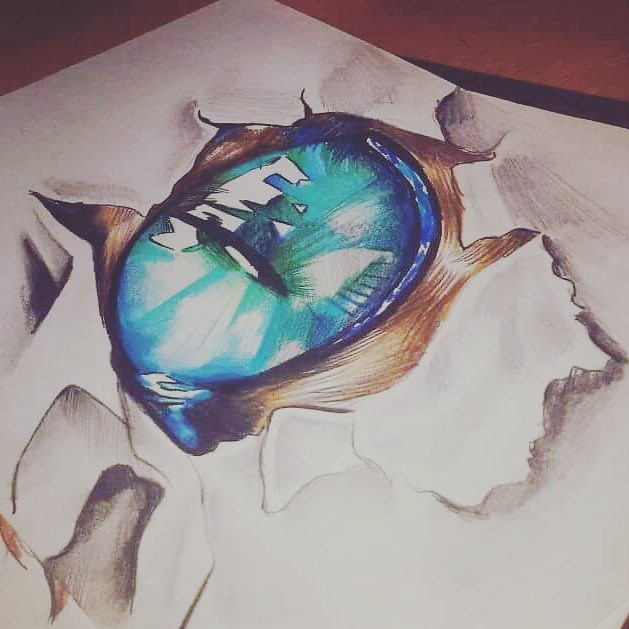This detailed caption describes a drawing of a cat-like eye in a nuanced manner:

"A meticulously rendered drawing of a cat-like eye, executed on off-white, light cream construction paper, laid on a surface partially visible as a dark brown faux wood color. The drawing, done primarily in pencil and colored pencils, showcases the eye's outer regions in a striking deep blue that gradually transitions into a vibrant turquoise, reflecting a green-blue hue. The pupil is a distinctive slit, characteristic of feline eyes, and includes an ambiguous reflection within it. The area surrounding the eye displays an array of jagged outlines and eclectic patterns composed of various brown tones, enriched with numerous squiggly lines and abstract shapes, adding a dynamic background to the central eye motif."